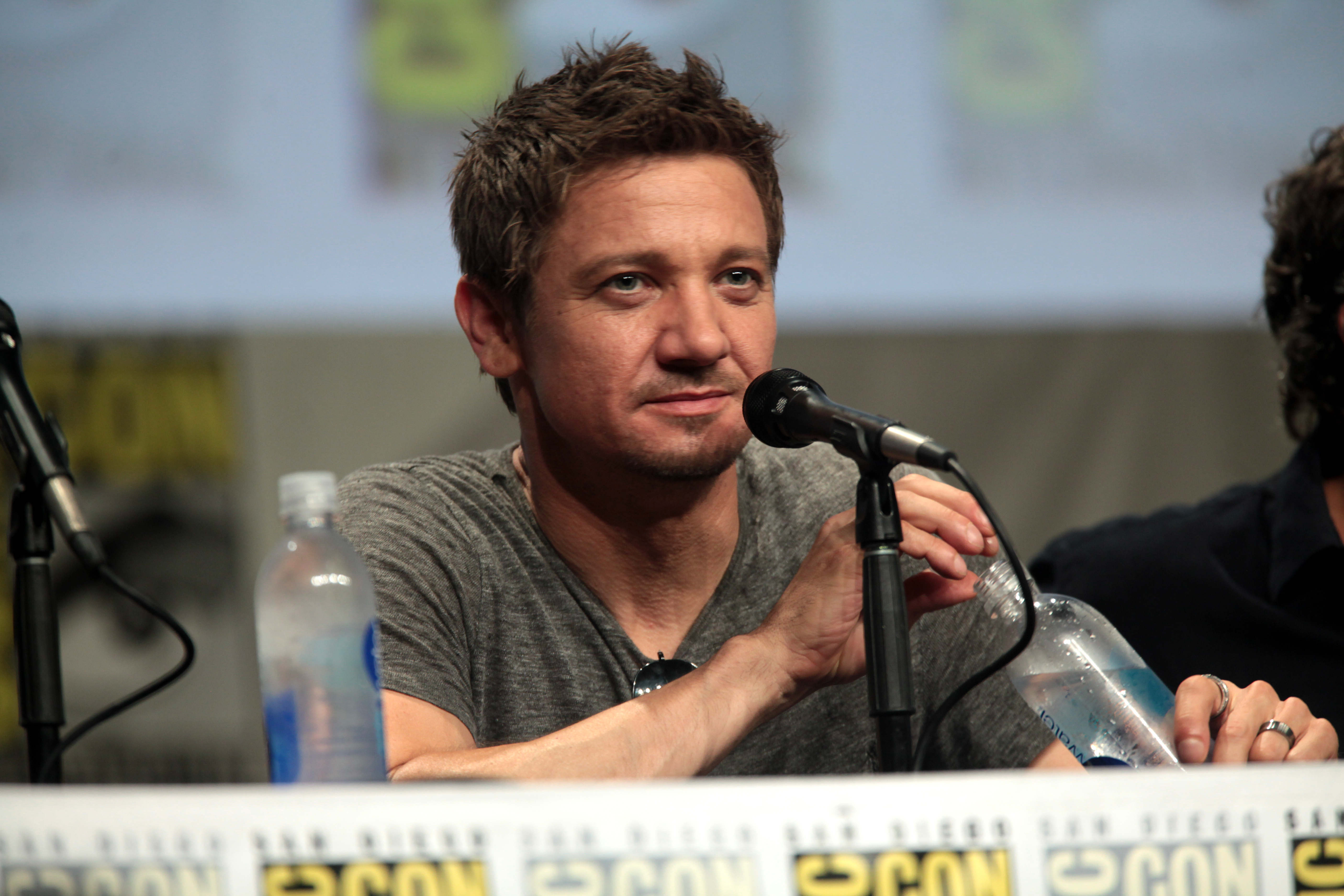In this image, a Comic-Con panel scene is vividly depicted. At the forefront, actor Jeremy Renner is seated at a white table adorned with Comic-Con logos. Renner, a white man in his forties or fifties, has short, slightly messy brown hair styled with gel, and he sports a gray, heather-gray v-neck with glasses hanging from the collar. He has a stubble goatee and is focused on the audience while handling a water bottle, either placing the cap back on or having just removed it. A microphone is positioned in front of him. Next to Renner sits another individual with black hair and a black shirt, with a microphone and another water bottle situated to their left. The background features a blurred screen with more Comic-Con logos, which are also displayed prominently on a banner at the table's base.